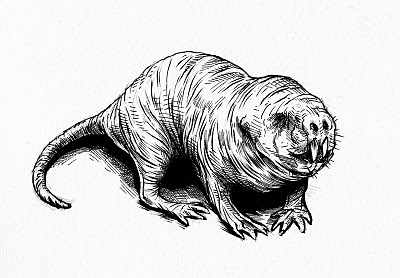This detailed black ink drawing, created on white paper, features a hairless, wrinkled skin mole-like creature prominently shown in a vertical head-on view but angled slightly to the side. The creature, resembling a naked mole rat, has no visible fur except for some potential whisker-like hairs on its face and possible small protruding hairs elsewhere. It has webbed feet with finger-like extensions and no apparent ears. Its facial features include two menacingly large teeth and two small holes in place of a nose, creating a sense of eeriness and life. The eyes are either scarcely visible or not visible at all. The illustration showcases much detail, particularly in the creased, textured skin and the claws, emphasizing the creature's peculiar anatomy.